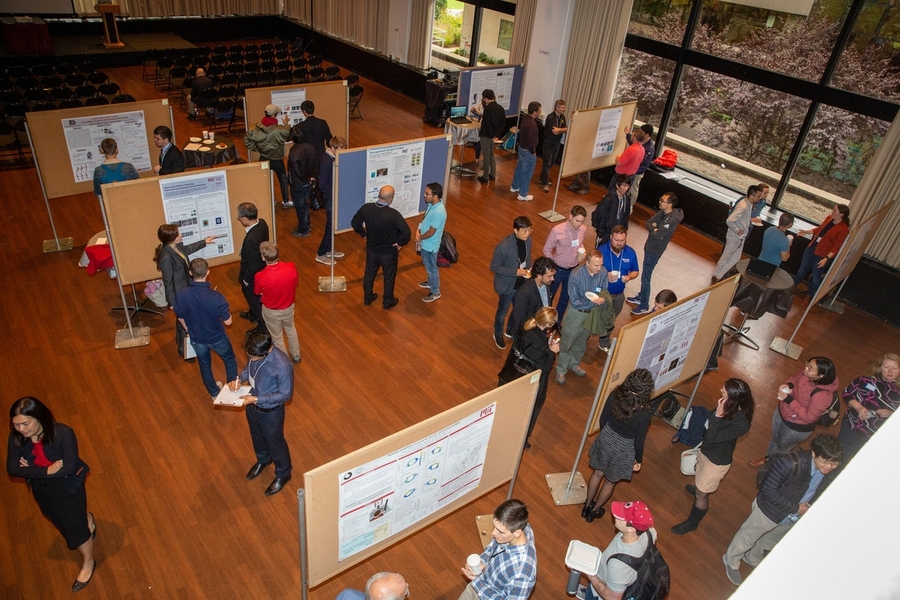The image captures a bird's-eye view of a bustling convention or fair in a large conference room with hardwood floors. The room is filled with people, many wearing name tags and some dressed warmly, indicating it may be cold outside. They are gathered around various informational displays mounted on cardboard stands, engaging in discussions about the presentations. On one side of the room, there are approximately 10 rows of chairs arranged neatly, presumably for an audience. Adjacent to these chairs is a small wooden podium on a platform, suggesting potential discussion panels or speeches. Large windows line the walls, revealing a wintry outdoor scene with snow-covered ground and woodsy surroundings. The room is well-lit, providing a clear view of the numerous attendees, some of whom carry backpacks and cups of coffee, immersed in the event's activities.